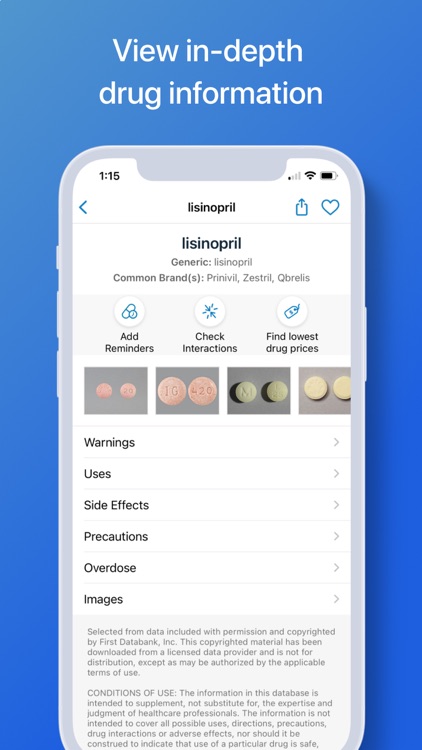**Caption:**

The image features a blue background with a prominent white cell phone illustration in the center. The phone screen displays a message: "View in-depth drug information." The drug highlighted is Lisinopril, also known by its generic name Lisinopril, and listed under common brands like Prinivil, Zestril, and Qbrelis.

The interface encourages user engagement by providing options to add reminders, check interactions, and find the lowest drug prices. The design includes four distinct sections, each with both front and back images of pills on a gray background – two pink, one green, and one yellow.

For additional information, clickable right arrow icons on the right side lead to detailed sections on warnings, usage, side effects, precautions, overdoses, and images.

At the bottom, there is a disclosure stating that the content is selected from data provided by First Data Bank, Inc. and is protected by copyright. It is highlighted that this information is licensed and should not be distributed beyond agreed terms. The database is meant to complement professional medical advice, not replace it.